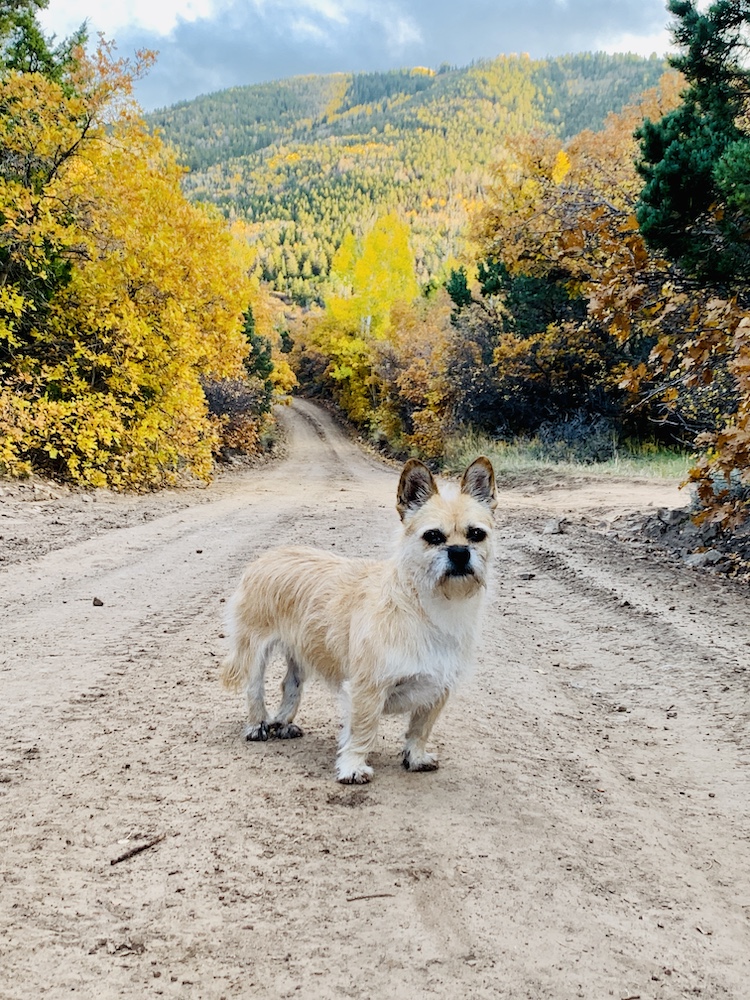This photograph features a small tan and white dog standing on a wide dirt road in the middle of a forest. The dog, which has short legs, a black nose, and short ears, is looking directly at the camera. Its fur shows a mix of white and various shades of tan or beige, with its face and back displaying more tan, while its neck and chest are predominantly white. The road, suitable for a car, stretches off into the distance, flanked by dense forests on both sides. The trees exhibit vibrant autumn colors, with hues of yellow, orange, and green, suggesting the season is fall. In the background, a large hill or mountain covered with tall, green trees is visible, enhancing the scenic beauty of the location. On the right side of the photo, there are some rocks and sticks scattered on the ground, adding a rustic touch to the natural landscape.